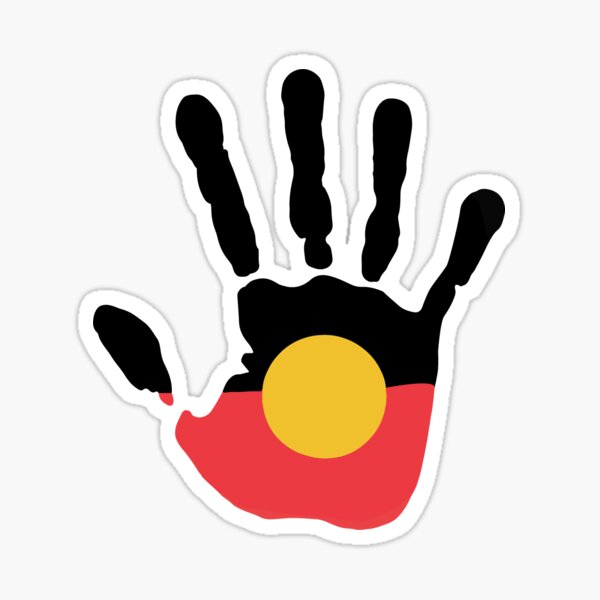The image displays a handprint with a striking color scheme and distinct design elements, set against an off-white rectangular background. The handprint features a solid white border that outlines the entire shape of the hand, including the thumb and four extended fingers. Each finger and the thumb are painted black, with a black section also coloring the upper part of the palm. Below this black area, the lower half of the palm transitions into a rose red color. In the center of the palm, overlapping the black and red sections, is a dark yellow circle, possibly resembling a sun. This design, marked by its bold colors and clear lines, resembles a stylized or perhaps primitive graphic artwork.